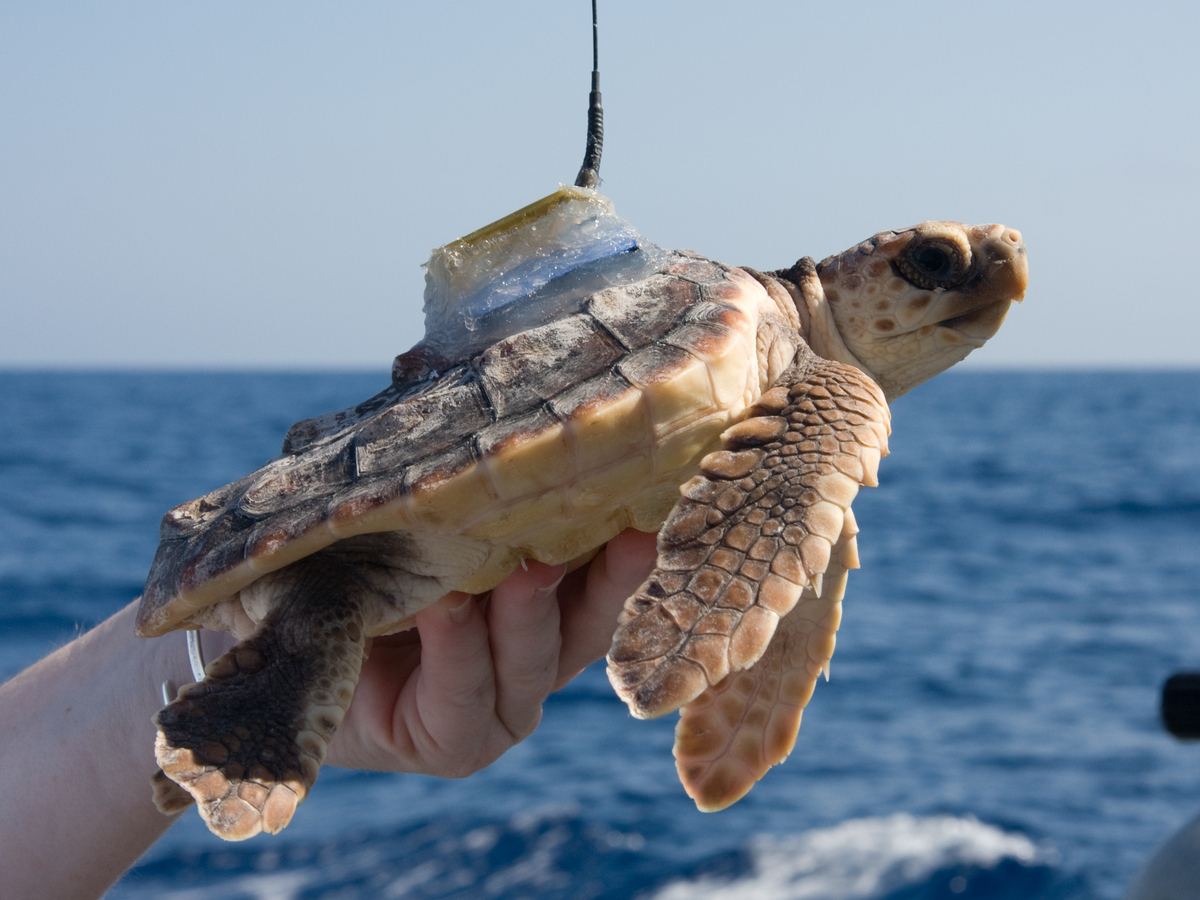In this image, a small sea turtle is prominently featured, held aloft by the hand of a white person. The scene is set against a breathtaking backdrop of a deep blue ocean stretching endlessly into a clear, cloudless sky, with the sunlight casting a warm glow over the scene. The turtle, centered in the frame, faces up and to the right, its large eye noticeable and inquisitive. Its shell is primarily brown and flat, adorned with a man-made device that appears to be glued on, contrasting its natural appearance. This device consists of a blue bottom, a dull yellow top, and a white, filmy, gel-like substance covering it, with a radio antenna protruding from the top. The turtle's flippers and head share the same brown hue as its shell, while its belly and throat display a dull yellowish-orange or cream color. The hand holding the turtle is close to the water, suggesting the photograph was likely taken from a boat.